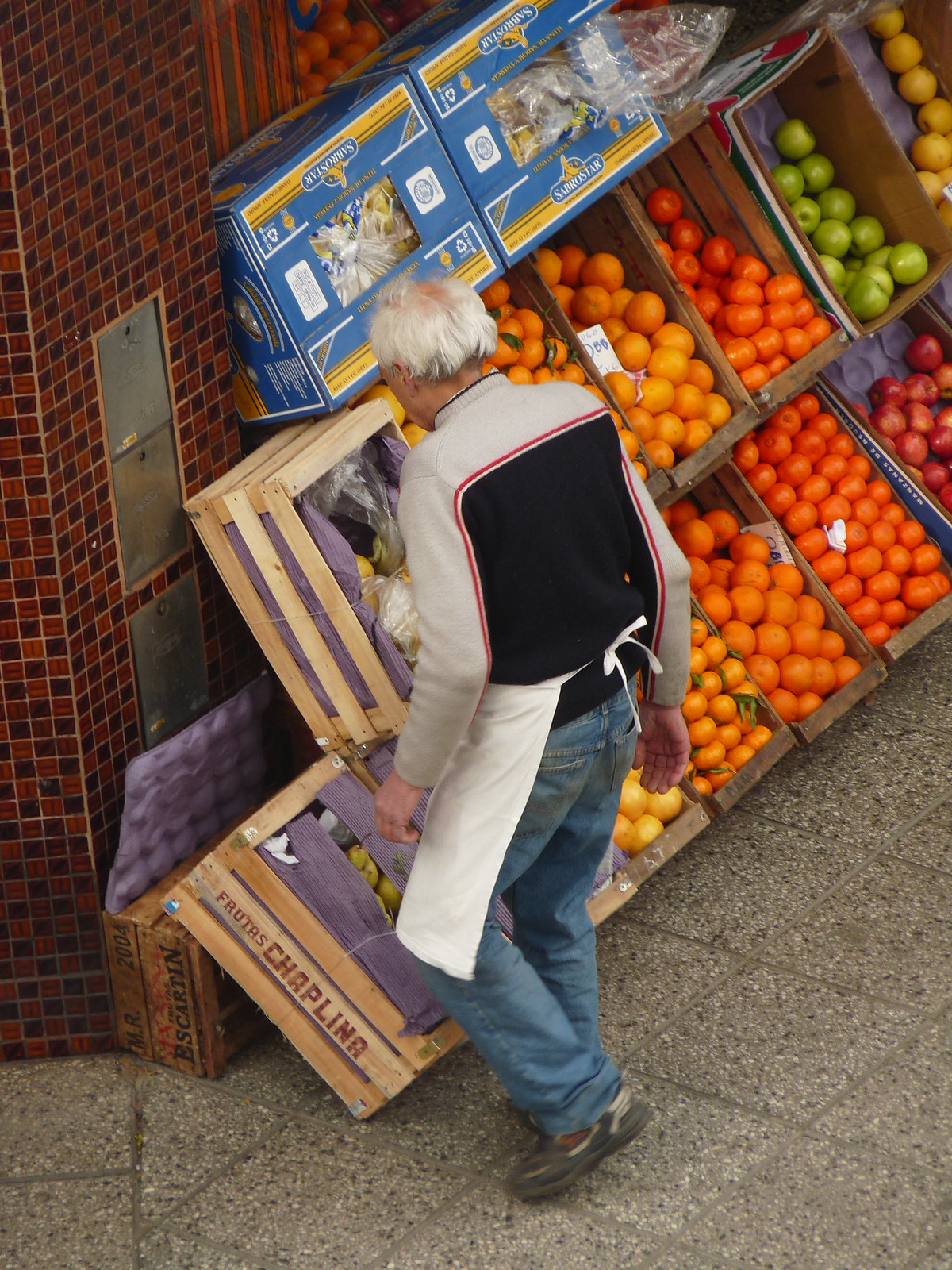This detailed color photograph, taken in portrait orientation, captures an outdoor fruit market scene. Positioned against a pattern of brick tiles, the setting features various fruits meticulously displayed in crates and cartons. Central to the image is an older man with long gray hair, a receding hairline, and wearing a white apron, a gray sweater with black accents on the back, and blue jeans. He is seen from behind, attentively gazing at the array of fruits. The fruits include green and yellow apples, oranges, tangerines, and lemons, with every crate brimming with colorful produce. Some crates are wooden with one marked "Frutas Chaplina," and a cardboard box labeled "Bascaritan 2000" is also visible. Additional closed crates are stacked on top, while open crates below contain fruits, possibly potatoes in purple wrapping, all arranged neatly along a pebble walkway.